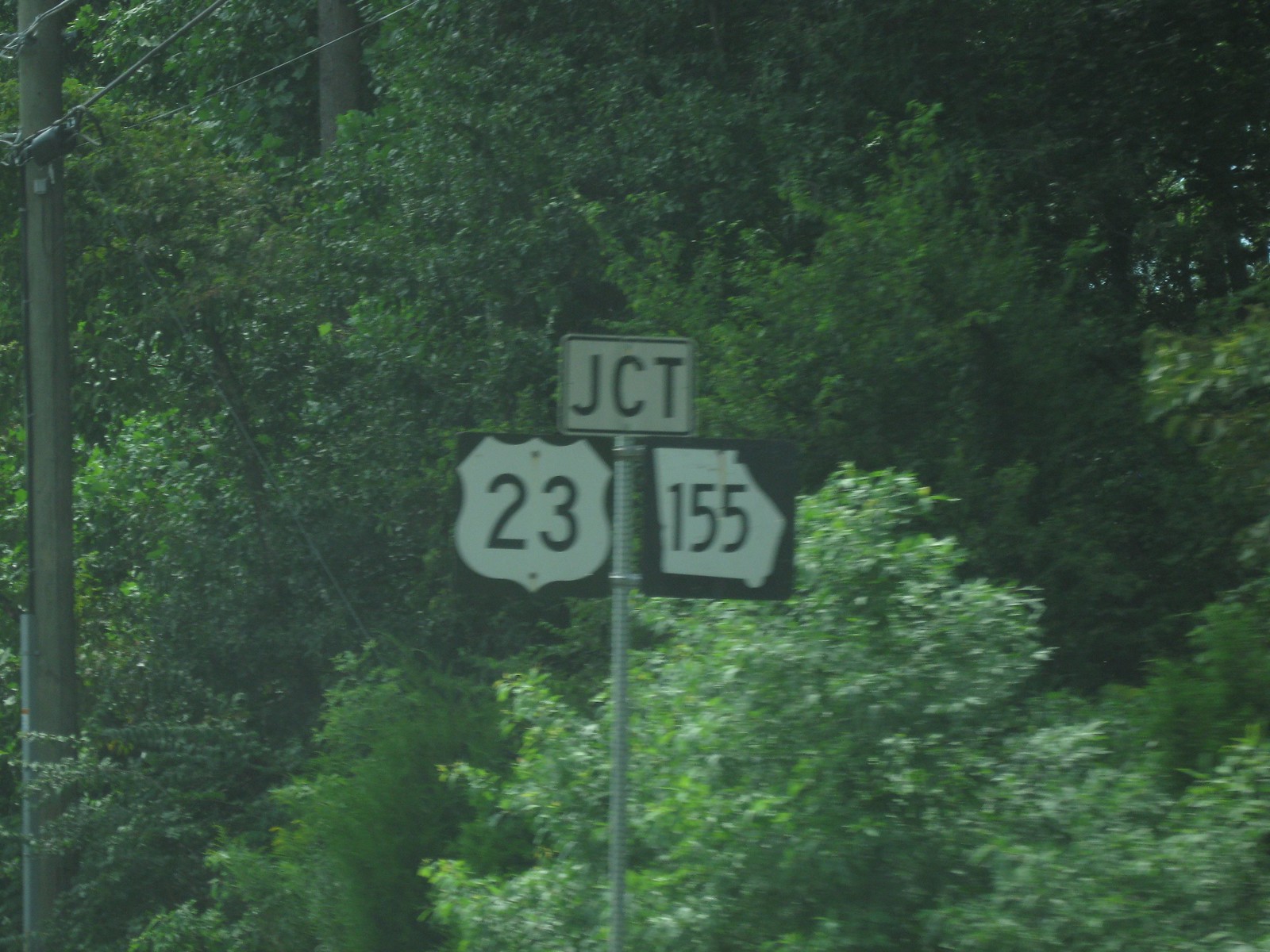A photograph captures the intersection of County Road 23 and State Highway 155, with a distinctive sign indicating "JCT" for junction. The state highway sign uniquely mimics the shape of Arkansas, adding a touch of local identity. Surrounding the junction, a serene landscape unfolds with clusters of lush trees and dark wooden power lines carrying numerous thick cables. The scene blends rural tranquility with subtle indications of civilized infrastructure.